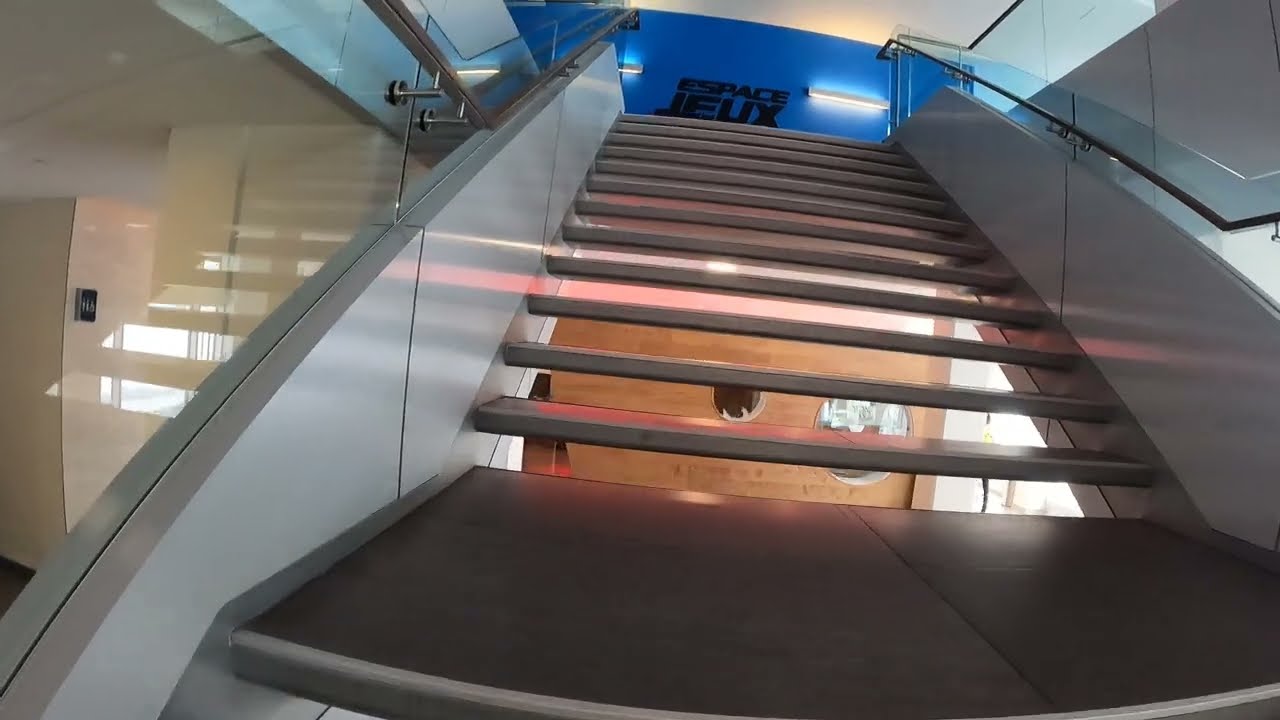The photograph captures a pristine stairwell leading up to a blue wall adorned with black lettering that reads "ESPACE JEUX," likely in French. The staircase features a dozen or so steps with silver treads and transparent risers, allowing a view of the brown wall below. The sides of the stairs near the bottom are framed by white panels that transition into clear glass balustrades and are capped with sleek silver handrails. Positioned centrally in the image, the stairs ascend towards the top, where the blue wall is subtly illuminated by discreet fluorescent lights. To the left, through the transparent sections, there are additional white walls, hinting at a well-maintained, modern building, potentially a hotel or a commercial space. The overall scene is captured from the bottom of the stairs, looking upward, emphasizing the clean, new look of the entire setting.